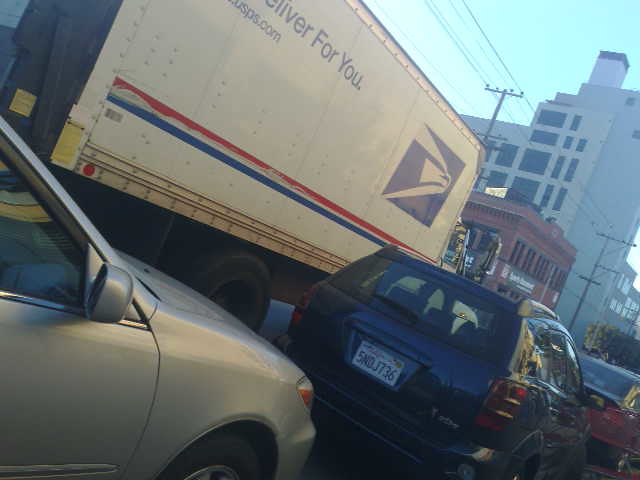In this image, we observe a scene of very busy traffic. The left side features a gray car partially visible, showcasing its rearview mirror and the upper part of its black tire. Ahead of this gray car is the back of a black SUV, with part of its right side also in view. Moving forward, there's a small visible portion of a red sedan, specifically its backside. To the left of these three vehicles, a large mail truck stands prominently. The truck is tall and white with horizontal red and blue stripes, displaying a blue logo at the top right corner and the text "Deliver for You, USPS.com" in blue lettering. One of the truck's tires is visible. In the background, a square-shaped building with black windows and brown color can be seen, surrounded by two large gray buildings. Above this bustling urban scene, the sky is a light blue.